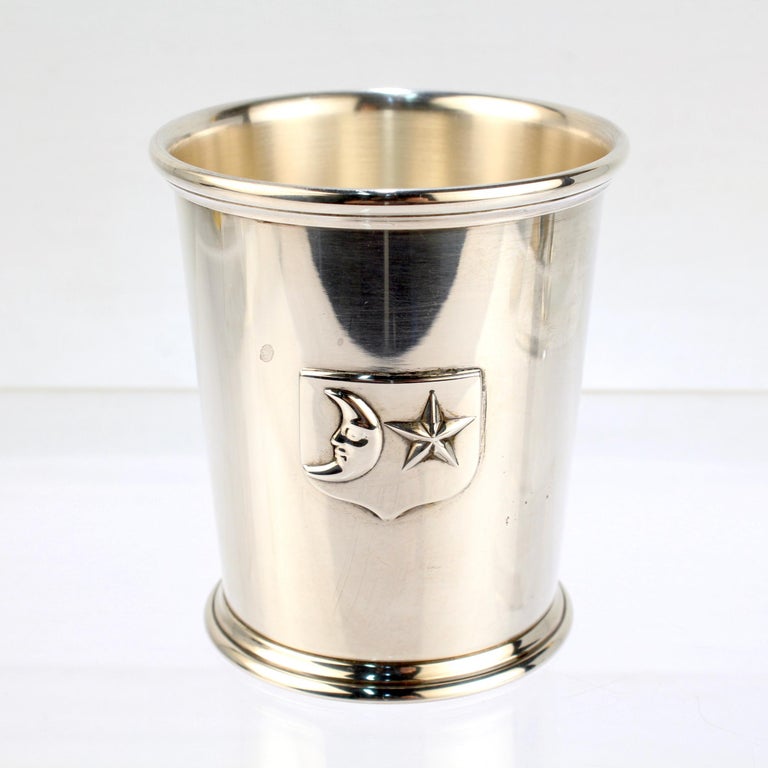This photograph features a polished stainless steel shot glass, centrally placed against a nearly flat white background with a faint gray line that could be either the side of a table or a shadow, making it difficult to determine the exact proportions of the object. The shot glass, characterized by a high polish finish, features two metal rims - one at the top and one at the bottom. Both the upper and lower rims are beveled, adding to its refined appearance. Prominently displayed on the front of the shot glass is a detailed emblem: a shield shape flanked by a crescent moon with a face on its left, and a Soviet-style five-pointed star on its right. The glass appears empty, and its surface reflects indistinct objects that suggest possible reflective surfaces nearby.